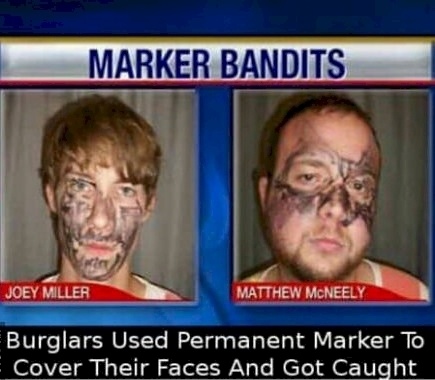The image appears to be a screenshot from a news segment titled "Marker Bandits," set against a dark blue background with a silver banner at the top bearing blue text. Centrally, the image features two photographs side by side. On the left, a young male, identified by white text on a red banner as Joey Miller, has brown hair and is wearing a blue and white striped shirt. His face is partially covered in black marker, mostly around his eyes, but not his nose or mouth. On the right is an older, heavier-set man named Matthew McNeely, also wearing a blue and white striped shirt. He has a full beard and black marker drawn over his cheeks, nose, and around his eyes, avoiding the mouth. At the bottom of the image, a black banner with white text reads, "Burglars used permanent marker to cover their faces and got caught."